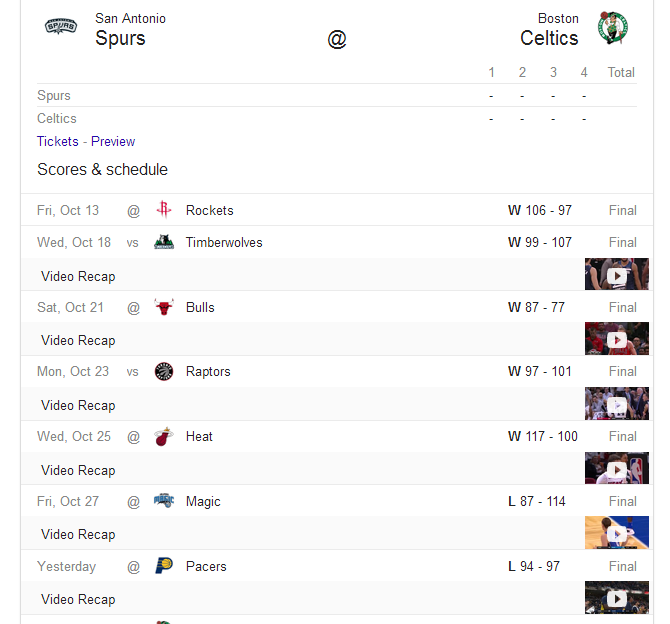The image displays a scoreboard for an upcoming basketball game between the San Antonio Spurs and the Boston Celtics. Positioned in the top left corner is the San Antonio Spurs' name, while the top right corner features the Boston Celtics' name. The scoreboard includes columns labeled for the first, second, third, and fourth quarters, although no scores are present yet, indicating the game has not started.

Below the main scoreboard, additional sections provide more information: tickets, a preview, scores, and a schedule. The schedule outlines previous games for the Spurs, detailing the opponents, game dates, and outcomes (win or loss). Each past game entry is accompanied by a video link for further details.